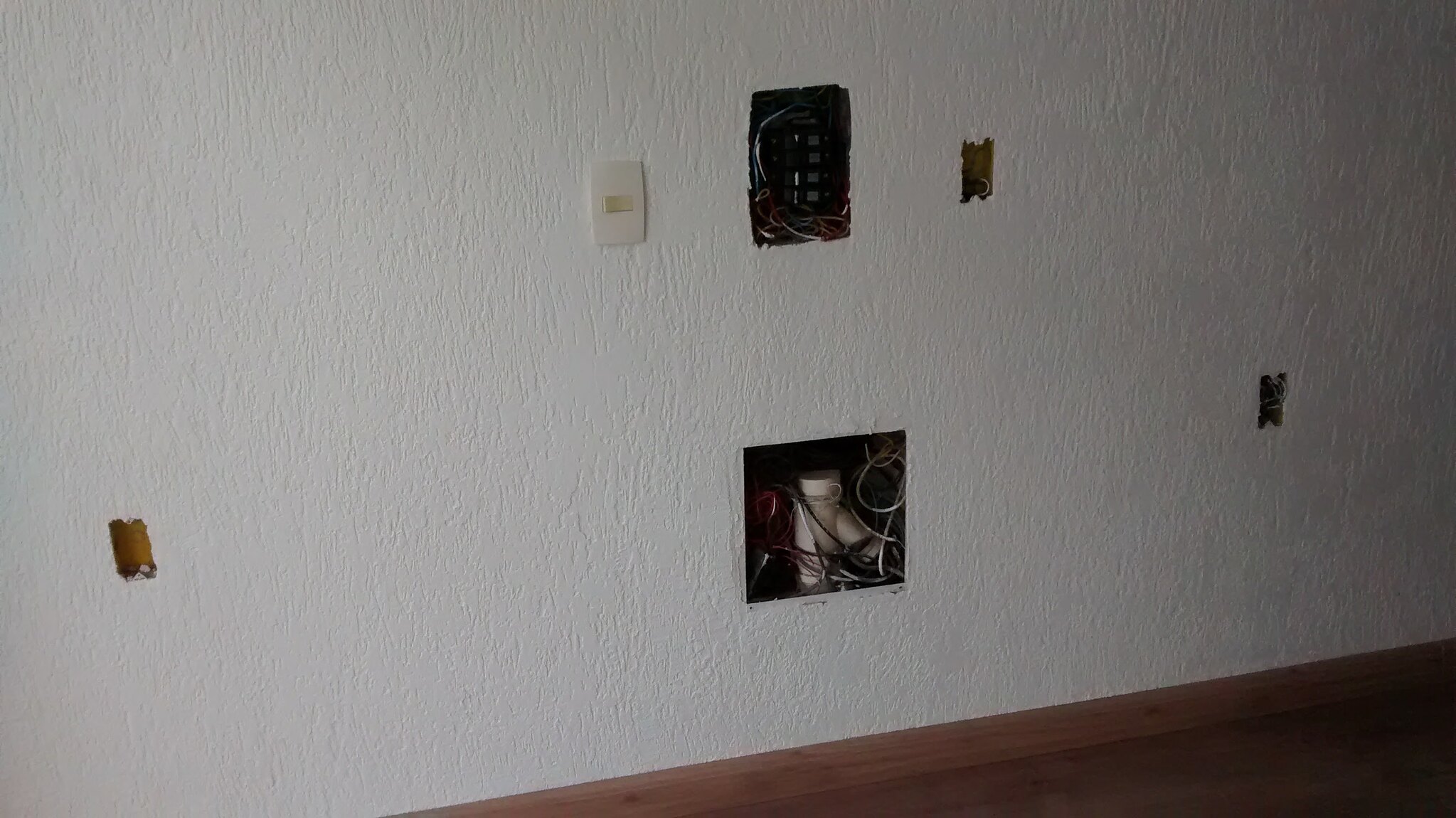The image depicts a white, textured wall characterized by several intentional cutouts meant for electrical fixtures. Most of these cutouts are rectangular, awaiting the installation of faceplates. However, one faceplate is already present at the left of the top center of the wall. This faceplate is off-white with gently curved edges and a central rectangular section that appears to be a rocker switch, which is more brownish in hue.

To the lower left, there is a small rectangular hole with a brown background, while a similar small rectangular hole to the lower right displays a black background with notches at the top and bottom. Another small, rectangular cutout with similar notches is positioned just to the right of the top center; this one has a mix of brown and black behind it.

Two larger holes are also notable: the upper one is a tall rectangle filled with multiple wires and a dark object featuring gray squares, obscured by shadows making it hard to identify. 

The largest cutout, at the lower center of the image, is square-shaped and houses a white pipe amidst numerous wires that are black, white, and possibly red in color. 

The scene is completed with a wooden trim at the bottom of the wall and a wooden floor, adding a touch of warmth to the otherwise industrial interior.